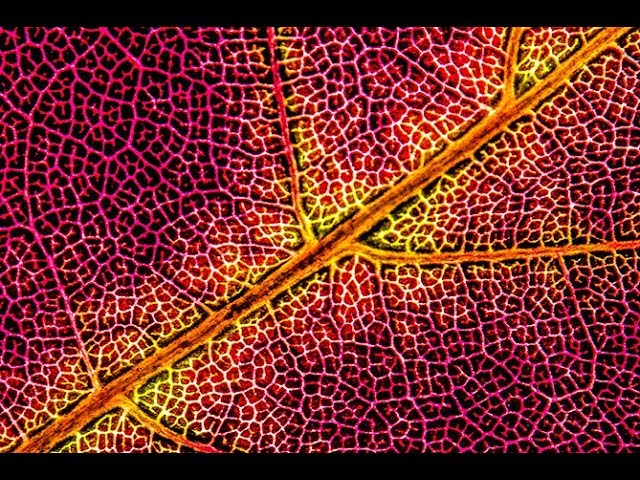This visually striking image presents a magnified view of a leaf under a microscope, emphasizing the rich and detailed structure of its veins. Dominating the composition, a gold-colored main stem runs diagonally from the bottom left to the upper right, branching off into smaller veins in several places—specifically, once in the middle and again near the top. These smaller veins exhibit a transition in color from gold to light purple on the left side, while maintaining their golden hue on the right. The central stem appears dark in the center, framed by a vibrant yellow halo. The backdrop showcases an array of cell patterns, with the right side adorned in deep purples and the left side tinged with light yellow accents. This vividly colored image—featuring shades of yellow, reds, blacks, and orangish hues—is cropped at the top and bottom, emphasizing its horizontal, landscape orientation. The intricate patterns and color transitions suggest possible digital enhancement, further accentuating the exquisite details of the leaf's anatomy.